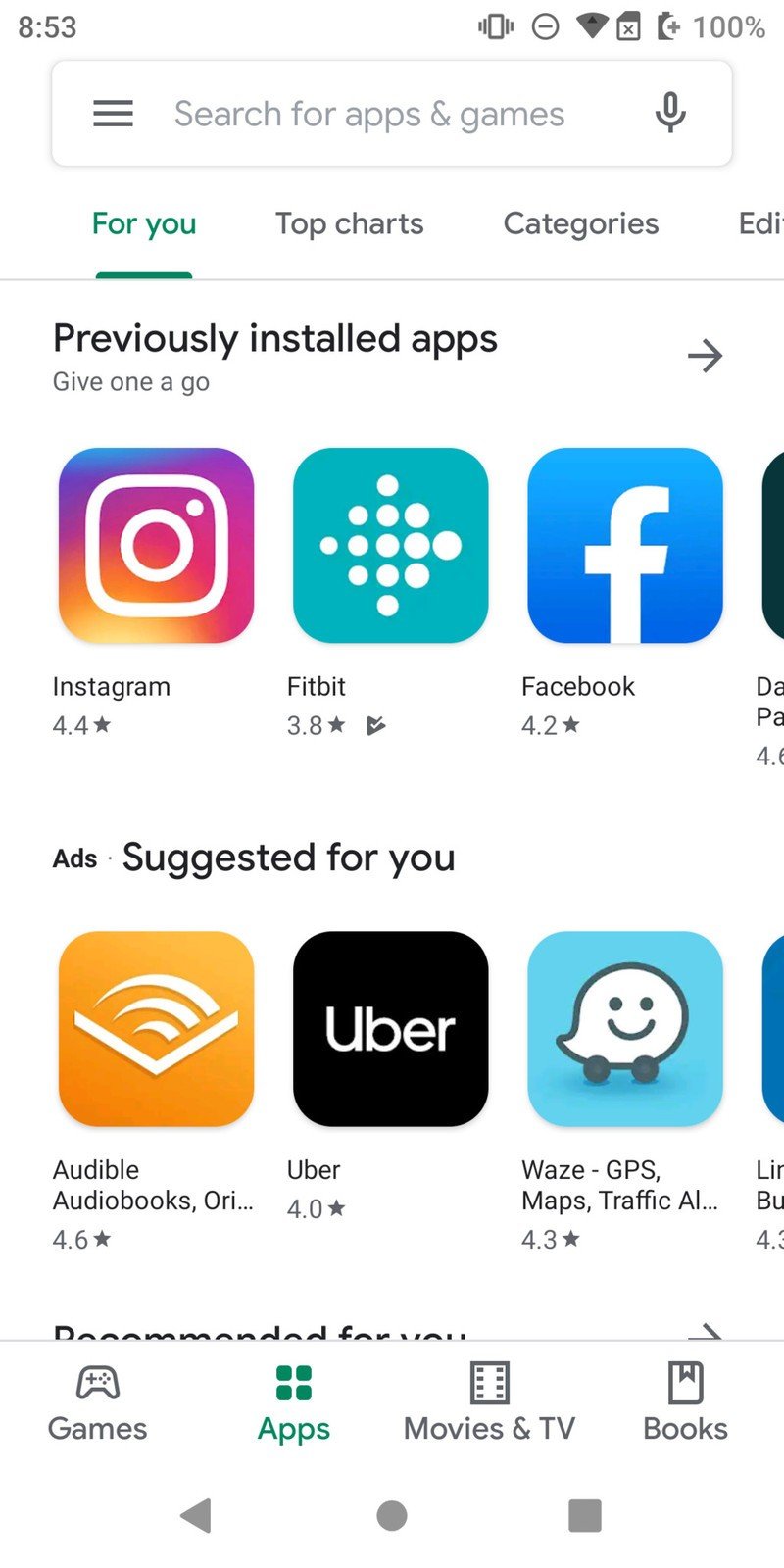This screenshot captures the Google Play Store on an Android device at 8:53 AM, as indicated by the time displayed in the upper left corner of the screen. The upper right corner shows the battery fully charged at 100% and a strong Wi-Fi signal. Prominently centered below the top bar is the Google Play search bar labeled "Search for apps and games," which is partially displayed. Directly underneath are the primary tabs: "For You," "Top Charts," and "Categories," with the "For You" tab currently selected.

Proceeding further down, under the "Previously Installed" section, the screenshot shows that Instagram, Fitbit, and Facebook are already installed on the device. Following this section is the "Ads Suggested For You" heading, showcasing three app suggestions: Audible, Uber, and Waze GPS & Maps, each accompanied by their respective icons.

Finally, at the very bottom of the screen, the navigation bar displays icons for various categories, including "Games," "Apps," "Movies & TV," and "Books," making it easy for users to explore different sections of the Google Play Store.